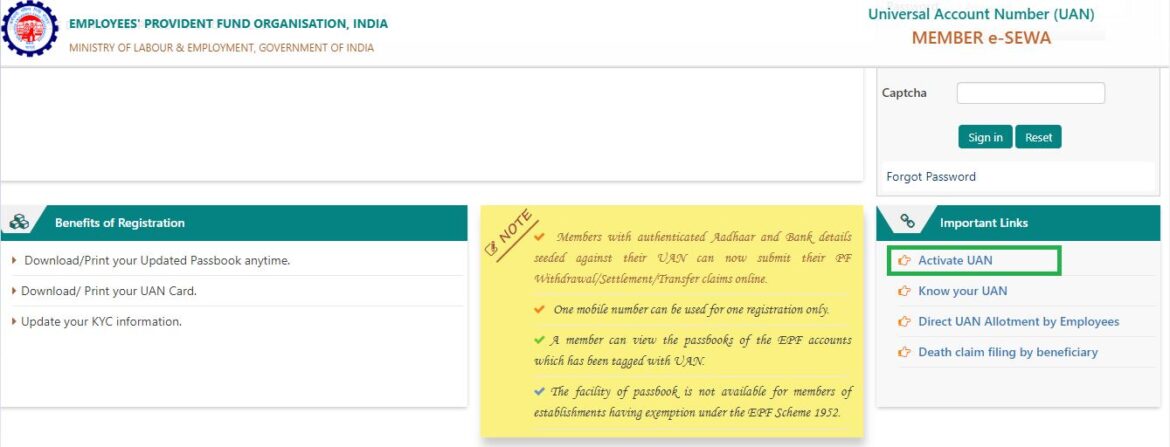This image showcases the homepage of the Employers' Provident Fund Organization (EPFO) website in India, affiliated with the Ministry of Labor and Employment, Government of India. In the upper left corner, a badge featuring the organization's logo is seen, although the image is slightly zoomed out. On the top right, prominently displayed, is the Universal Account Number (UAN) portal, labeled with "Member E-Sewa." Below this, the right column includes a CAPTCHA field along with "Sign In," "Reset," and "Forget Password" options. 

Towards the lower right, there is a section titled "Important Links" with several options listed, including "Activate UAN," highlighted by a green rectangular box, "Know Your UAN," "Direct UAN Allotment by Employees," and "Death Claim Filing by Beneficiaries."

At the center of the page, a yellow notepad-style notice informs members that those with authenticated Aadhaar and bank details linked to their UAN can now submit their Provident Fund withdrawal, settlement, and transfer claims online. Additional details include:
- A red checkmark noting that one mobile number can be used for only one registration.
- A green checkmark indicating members can view the passbooks of EPF accounts tagged with their UAN.
- A blue checkmark stating that the passbook facility is not available for members of establishments exempted under the EPF Scheme of 1952.

Finally, in the bottom left section, benefits of registration are listed in green. These include the ability to download and print updated passbooks, UAN cards, and to update KYC information.